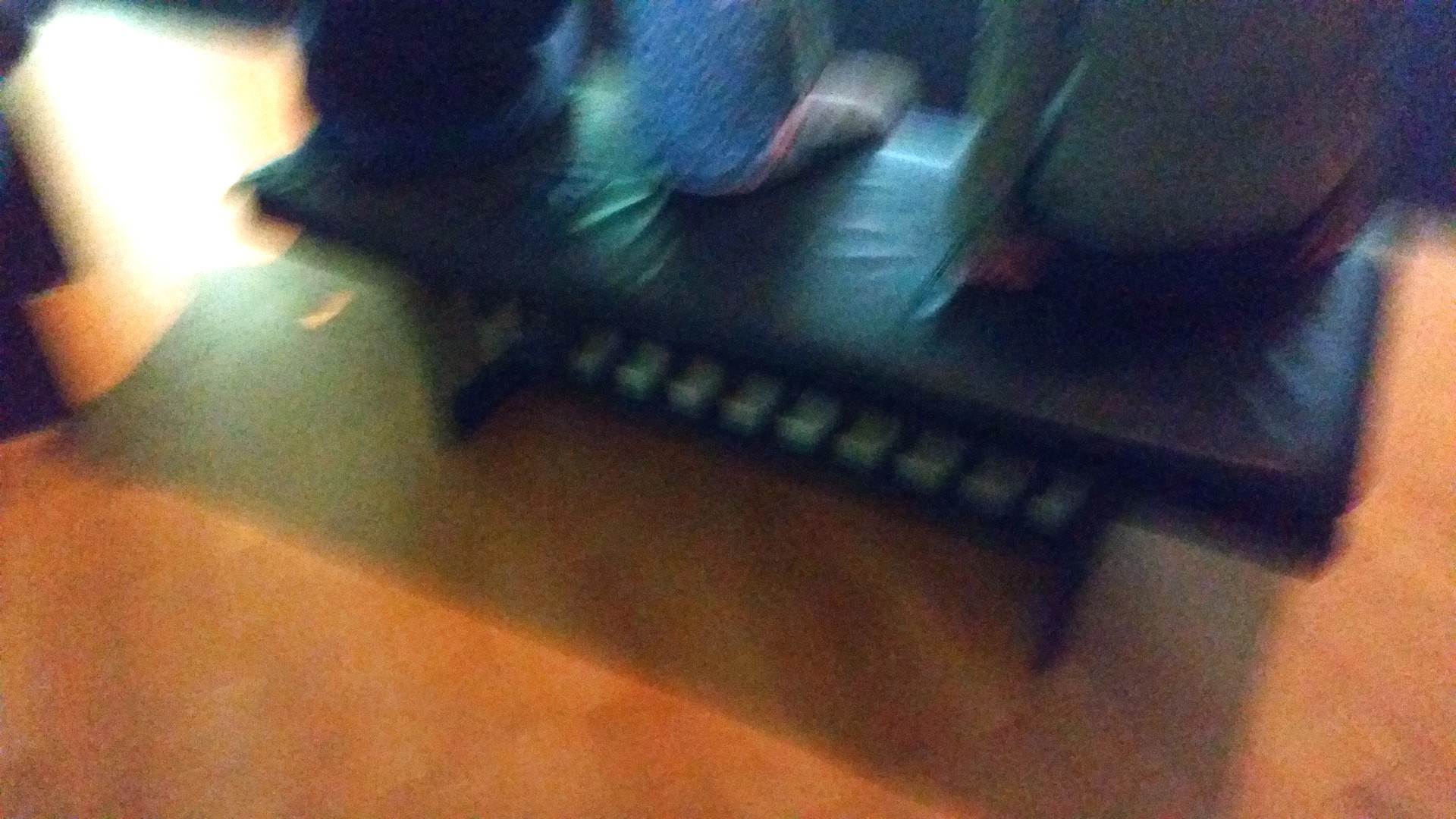The image is a blurry and out-of-focus scene featuring a rectangular bench with three people sitting on it, cut off at the torso or head, on a light orange-tan floor. The bench, which has a black leather-like cushion and a small black base, seems to have a detail resembling piano keys near the bottom. From left to right, the first person, likely a man, wears a light green long-sleeve shirt and black pants, with one hand balled into a fist resting on the bench. The second person, possibly a child, is dressed in a light blue shirt and white pants. The third person is in a black shirt and blue jeans, sitting with hands behind their back. Light shines through, casting the bench's shadow onto the floor, adding more depth to the setting.